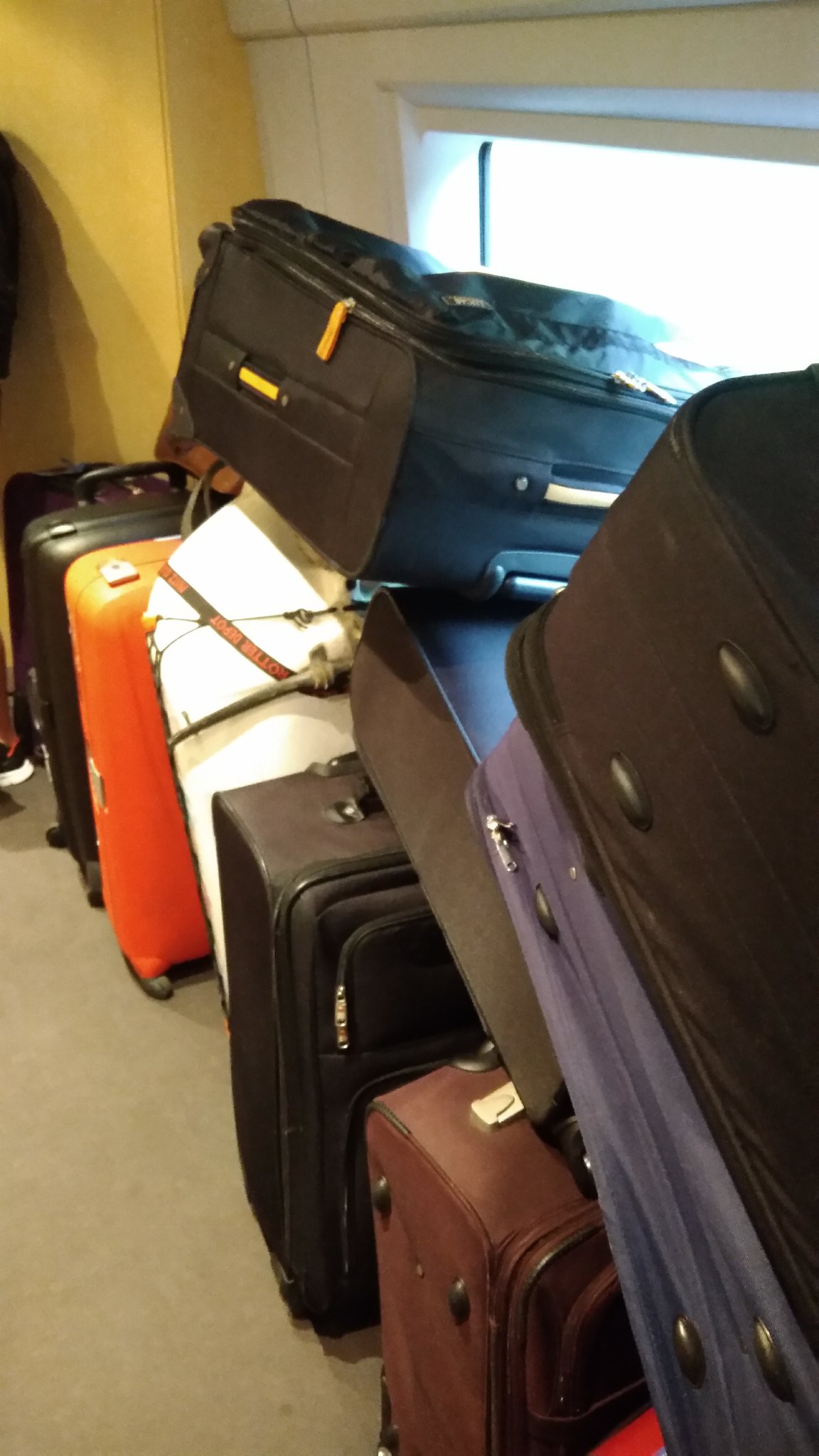The photograph showcases a haphazardly stacked pile of luggage, making it difficult to discern whether the setting is inside a vehicle, a building, or possibly a cluttered space like an attic. The suitcases are positioned against a yellow wall and a window with a white frame, situated on a beige or light brown floor. The luggage arrangement features around ten pieces in total, with a bottom row of five standing upright on their wheels and another layer of four laid horizontally across. The color palette of the suitcases includes black, orange, white, brown, bluish, gray, and purple. No labels are visible on the bags, leaving their ownership unclear. Notably, a black suitcase with white trimming or zippers is prominently positioned near the window.